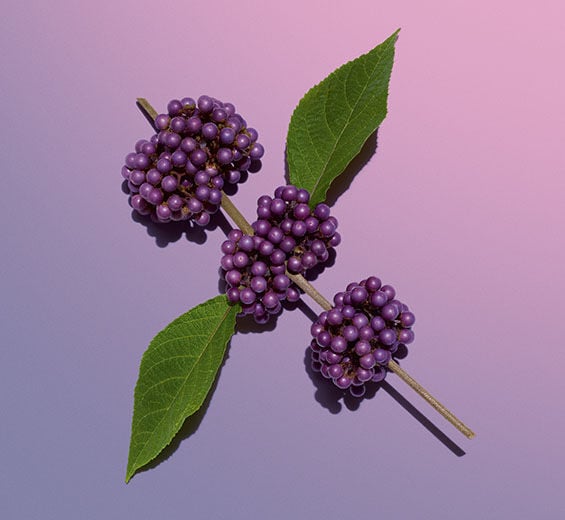The image depicts a light brown stem, possibly a skewer or stick, adorned with clusters of purple beads designed to resemble grapes, though these are unnaturally colored and positioned. There are three distinct clusters of beads, each mimicking grapes with varying sizes similar to BB pellets, making the largest cluster at the top of the stem, the middle one slightly smaller, and the bottom one the smallest. Two green, football-shaped leaves with jagged edges sprout from the middle cluster, positioned awkwardly. These leaves cast a dark gray shadow against a light purple and pink gradient background, contributing to the overall artificial and cheesy appearance.